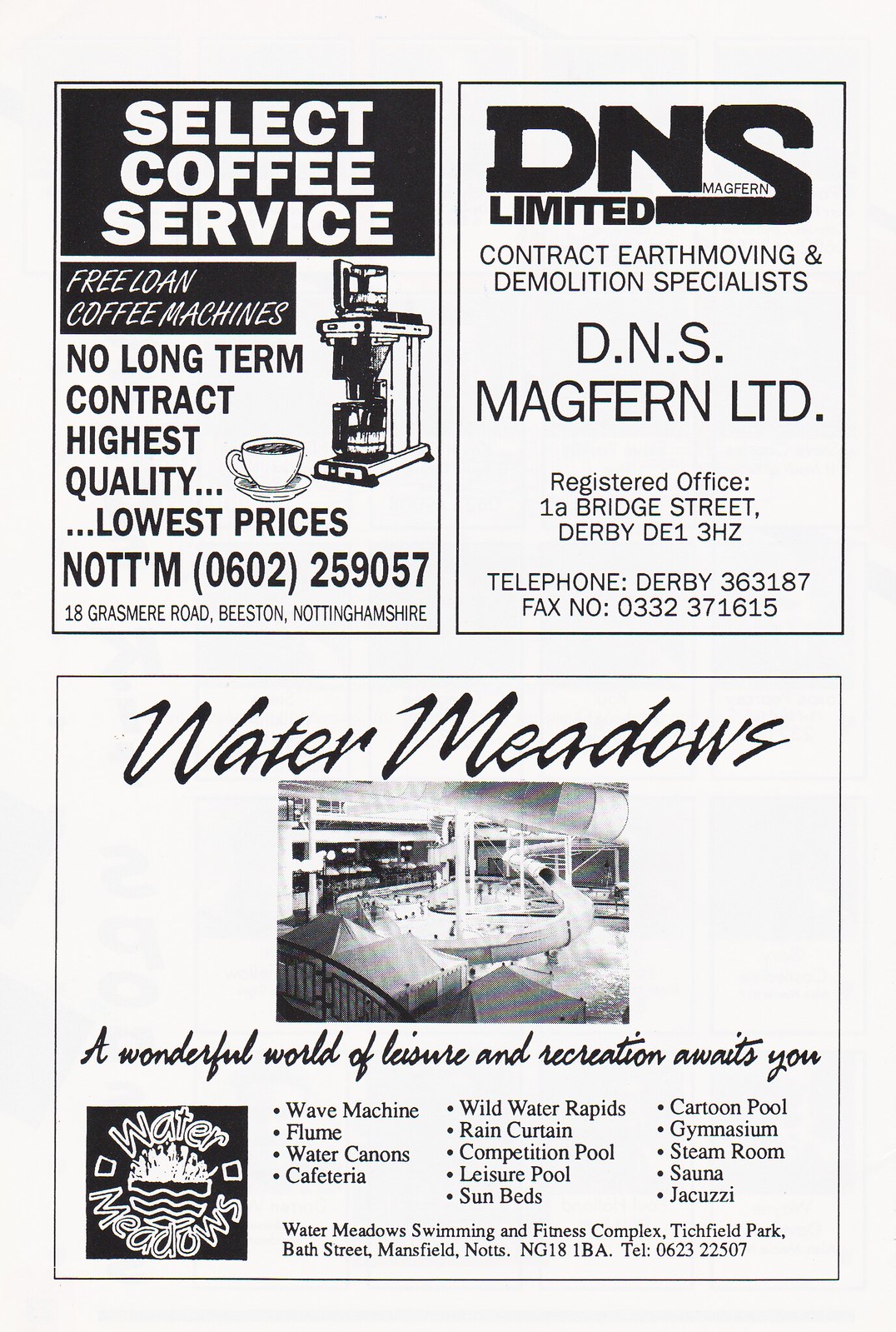This black-and-white page, reminiscent of a program or magazine ad layout, features three distinct advertisements. The top half is divided into two equal portrait-oriented sections. The left section promotes Select Coffee Services, showcasing a line art drawing of a coffee machine with a cup beside it, and highlights their offerings: Free Loan Coffee Machines, No Long Term Contract, Highest Quality, and Lowest Prices. The company's address is noted as 0602 Grasmere Road, Beeston, Nottinghamshire, and includes a contact number, 25905718. To the right, an ad for DNS Limited, Contract Earthmoving and Demolition Specialists, details services with the name DNS Magfern Ltd. prominently centered. Their registered office address is 1A Bridge Street, Derby, DE1 3HZ, along with telephone number Derby 363187 and fax number 0332371615.

The lower half of the page is dedicated to Water Meadows in a landscape-oriented half-page ad. The headline in script font reads, "Water Meadows," above a photograph of an indoor water park featuring a slide. The tagline, "A wonderful world of leisure and recreation awaits you," accompanies a comprehensive list of amenities, including a Wave Machine, Flume, Water Cannons, Cafeteria, Wild Water Rapids, Rain Curtain, Competition Pools, Leisure Pools, Sun Beds, Cartoon Pool, Gymnasium, Steam Room, Sauna, and Jacuzzi. The bottom left corner features the Water Meadows logo, while the bottom right provides the address: Water Meadows Swimming and Fitness Complex, Titchfield Park, Bath Street, Mansfield, Knotts, NG18 1BA, with a telephone number, 0623-225-07. The overall design is sleek and functional, emphasizing clarity and organization.